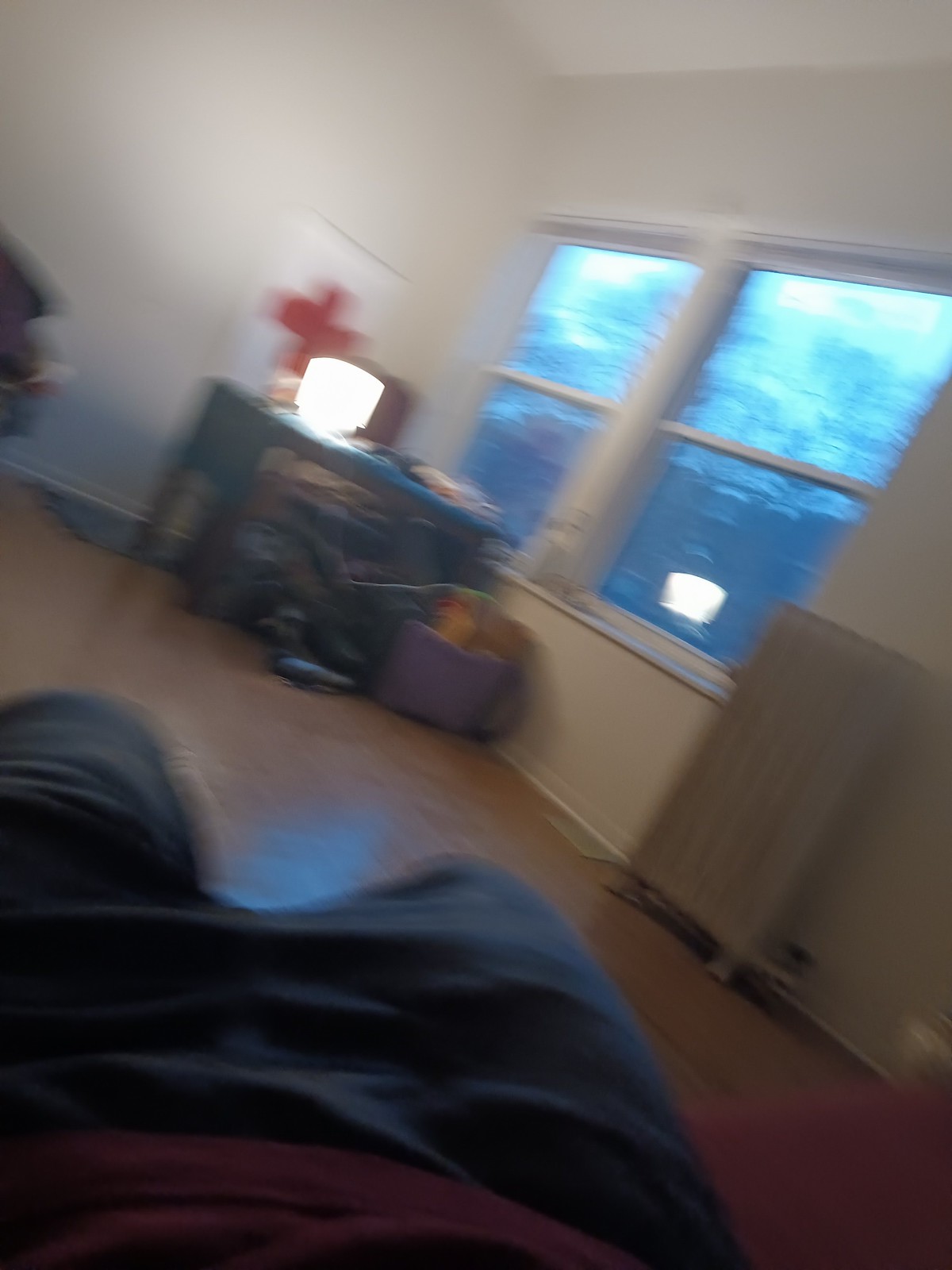This image captures a motion-blurred, low-quality photograph taken inside an apartment room, likely during the late afternoon. The camera shake is evident, making the entire scene appear blurry. In the bottom left of the frame, the lower torso and legs of the person taking the photo are visible. To the right, there is a radiator mounted against the wall beneath two adjacent windows, through which soft sunlight filters in. A desk with an illuminated lamp sits nearby, and a red-hued poster or picture hangs on the wall. The room has a wooden floor, but other details are obscured due to the poor image quality.